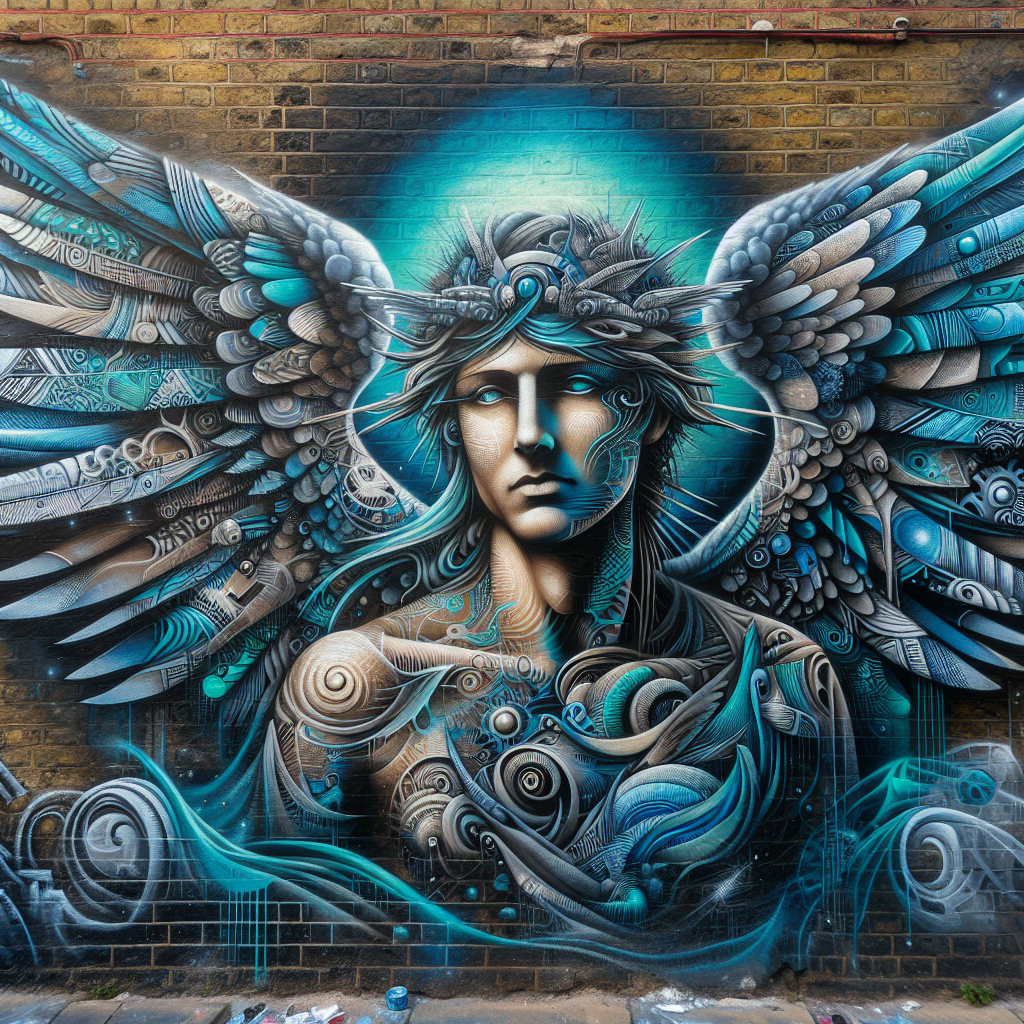The mural on the light yellow brick wall features a striking, somber-faced figure that resembles an angelic or mythological entity. The figure's hair is a mixture of gray and teal, crowned with an elaborate headpiece adorned with gray spikes in all directions. Their piercing blue eyes lack pupils, giving them an ethereal quality, and their face and upper body up to the pectorals are portrayed. The neck and one shoulder feature intricate teal-colored lines and swirls. 

Extending from behind the figure are large, detailed wings with feathers in shades of white, teal, blue, and hints of brown, creating a sense of movement as they spread upwards and outwards. The background around the figure is a radiant light that transitions from a bright white above the head to a more teal hue as it disperses. Among the decorative elements, abstract swirls and lines in similar teal and blue colors accentuate the design, creating a cohesive and vibrant aura around the figure. 

Below the mural, the sidewalk appears littered, and remnants of paint suggest ongoing or unfinished artistic work. Overall, the mural’s intricate designs and color palette of teal, gray, blue, and white lend it a captivating and almost mystical appearance, resembling a Greek statue merged with angelic symbolism.